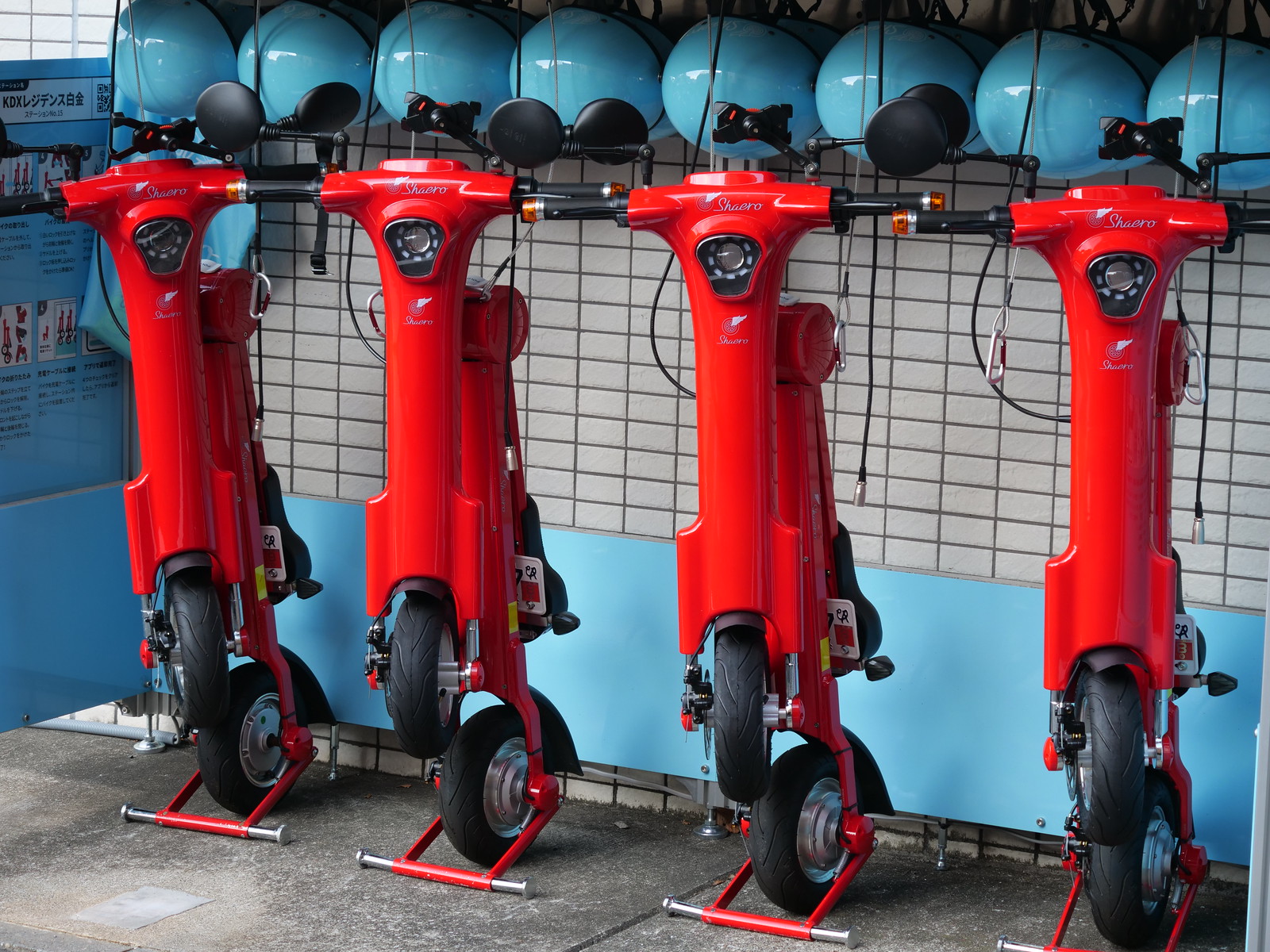In this sharp, color photograph taken in a landscape orientation, the central focus is on four red electric e-scooters, collapsed and folded up, standing neatly on their single kickstands. Each e-scooter features black plastic grip handles and small mirrors extending from one side of the handlebars. Between the handlebars, a circular lens, potentially for a light, is prominently displayed, enhancing the functionality and sleek design of the scooters. They are marked with the brand name "SHERO" in silver text. In the background, the image showcases aqua blue helmets with black straps and metal buckles hanging in a row against a netting on the wall, providing necessary safety gear for riders. The setting appears to be a vehicle workshop, evidenced by the rectangular white tiled walls interspersed with a light blue panel that seems to be partially detached. A sign on this panel, featuring white banners with black text, adds to the industrial ambiance of the scene.